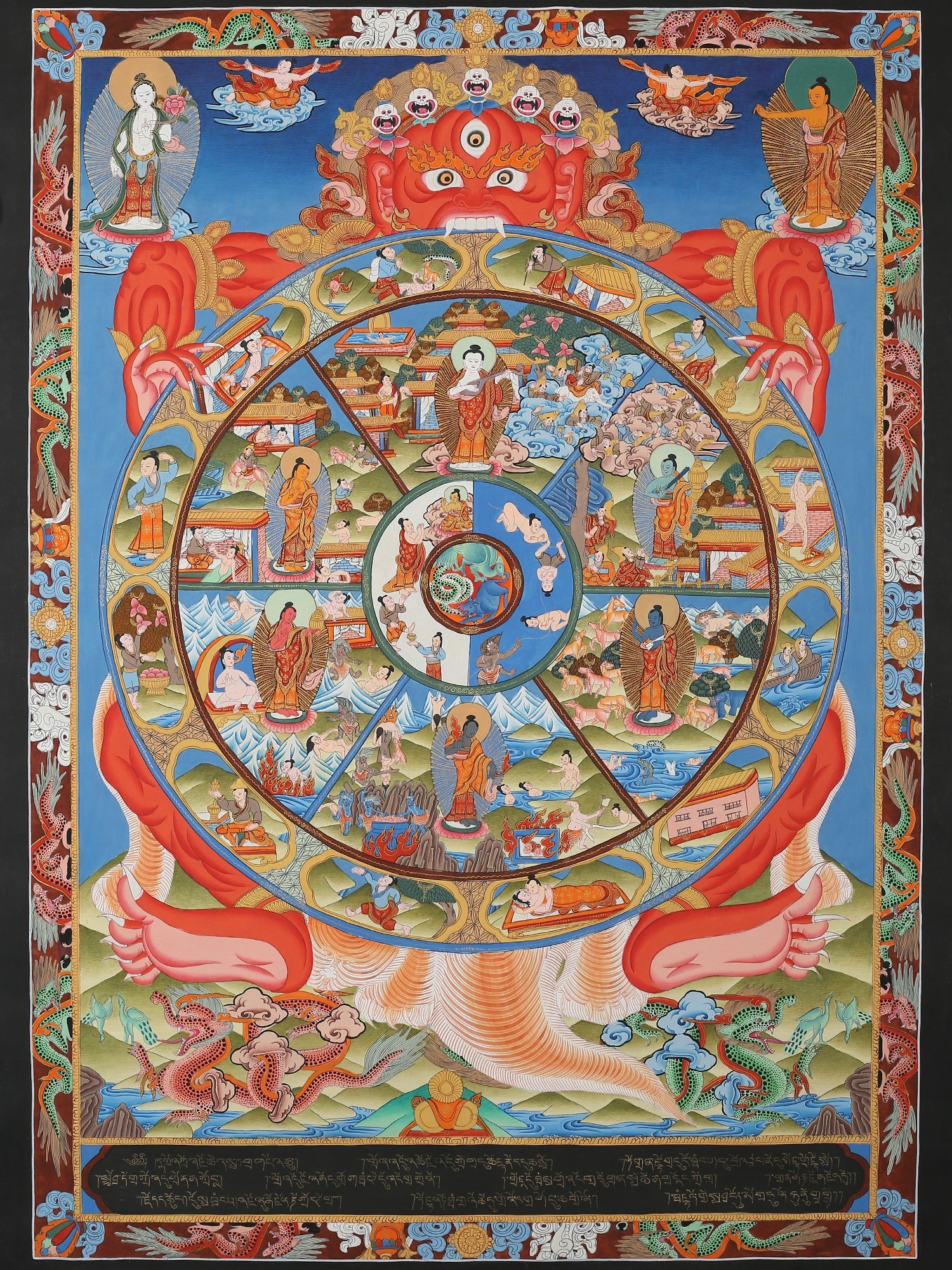This meticulously detailed piece of art, oriented vertically, captures the essence of traditional Eastern Asian or Indian Hindu styles, possibly reflecting the spiritual tenets of Buddhism or Hinduism. The intricate design centers around a vibrant circle divided into six segments, each depicting scenes of life, believed to feature a Buddha-like figure or other saintly characters dressed in traditional Asian attire with halos and wings, suggesting their ethereal or divine nature. 

Surrounding this central circle is a striking red demon-like figure with long toenails, a tail, extended claws, three eyes, and snakes for hair, reminiscent of mythological or religious symbolism. This menacing figure appears to bite into the circle, further accentuating the mystical and philosophical themes of the artwork.

The border is rich with ornate, multicolored dragons and includes various elements such as scrolls, fish, and pots, all set against a burgundy background. The art is framed by a combination of blue and black with a gold border. At the bottom, there's indistinct writing, adding another layer of mystery and depth to the piece. The detailed depictions reflect both cultural and philosophical aspects, making this artwork a profound representation deeply tied to Asian or Indian heritage.